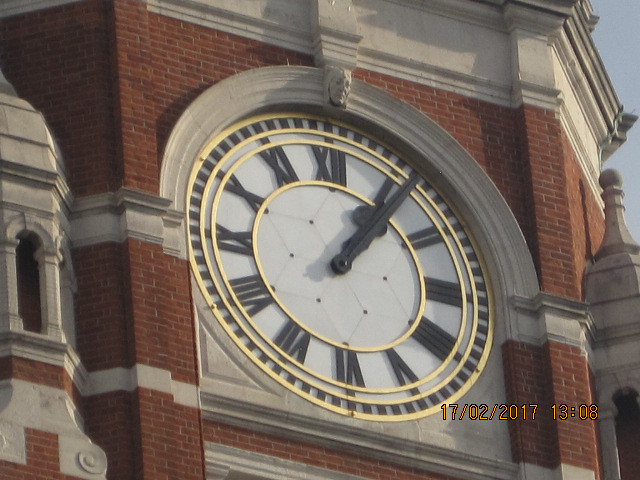This photograph showcases an imposing government building or significant establishment characterized by its grand red brick construction. The structure features ornate sculptures and intricate architectural details typical of governmental edifices. Dominating the composition is a large central clock with elaborate gold and bronze embellishments, displaying charcoal gray numbers. Just above the clock, there is an intricately sculpted face, adding to the building's almost gothic aesthetic despite its relatively modern construction. A timestamp on the photograph indicates it was taken on February 17, 2017, at 13:08, though it slightly mismatches the clock’s displayed time by approximately three minutes. In the top right corner, a sliver of the sky is visible, emphasizing the building’s towering presence.